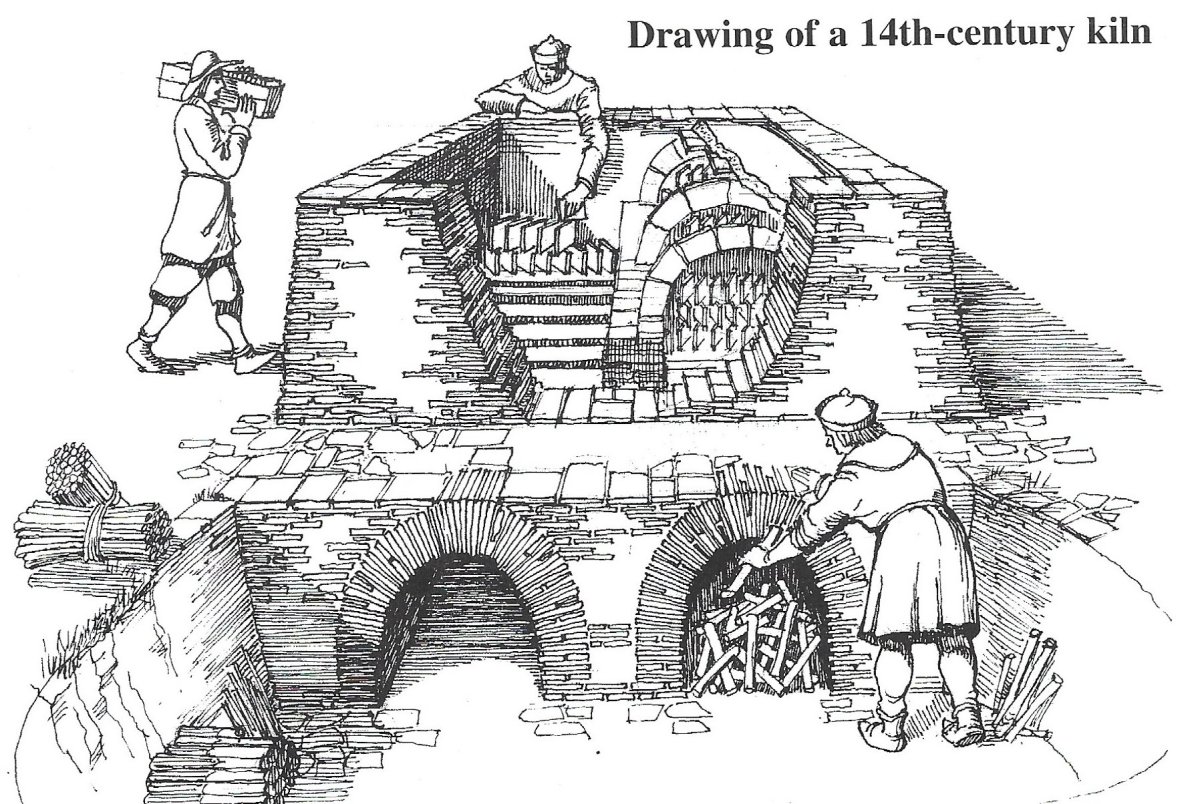This black and white penciled drawing depicts a detailed cutaway view of a 14th century kiln labeled at the top right with the text "Drawing of a 14th Century Kiln". The kiln is constructed into a hillside requiring access through lower ground to feed the fire from the bottom. The drawing is divided into two main sections.

In the upper section, a man can be seen standing behind the kiln on the left, visible from the chest up, reaching his left arm into the structure to arrange what appear to be tiles or bricks. To the right of him inside the kiln, there are semi-circular arches supporting the structure. In the foreground, the kiln has a stone façade with the right side sheared off, revealing the interior workings of the kiln and another open stone front creating a compartmentalized look.

In the lower section, there is a path in front of the kiln. Beneath this path, the kiln extends downward into a lower chamber accessed through two arched openings. The left arch has wooden sticks stacked inside, and a man on the right side is seen inserting additional wood into the right archway, with more pieces stacked nearby. The walls of this lower chamber show several vertical stacks of bound wood, indicating a storage area for the kiln's fuel. The structural composition of the kiln clearly shows it is built from a mix of stone and brick materials to withstand high heat.

The entire scene is brought to life by the detailed depiction of men engaged in the process of operating the kiln, dressed in period-appropriate long jackets, shorts, shoes, and socks with various types of hats, adding context and depth to the historical diagram.